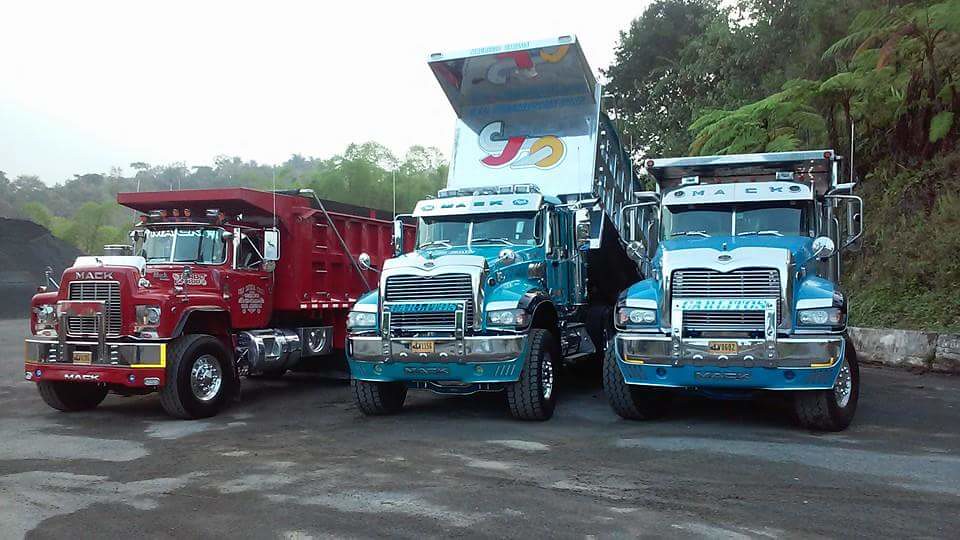This outdoor color photograph captures a trio of vintage Mack dump trucks parked on an asphalt parking lot. The scene is framed by a lush green landscape with trees on either side and a small hill adorned with foliage to the right. The sky above is a bright white, giving the impression of a cloudy day. 

The trucks, viewed primarily from the front, are distinguished by their vibrant colors and apparent upkeep. The leftmost truck, a striking fire engine red Mack, is slightly turned to show its side. The other two trucks, positioned centrally and to the right, are a matching baby blue. Notably, the central blue truck has its metallic dump bed elevated, revealing a logo with a white "C," a pink "J," and an inverted yellow horseshoe-like shape.

The parking lot's surface is a mix of dark and light gray, adding texture to the foreground. Behind the trucks, a concrete wall demarcates the end of the parking area, blending with the natural greenery. The overall composition emphasizes the trucks' substantial, heavy-duty nature against the serene, verdant backdrop.